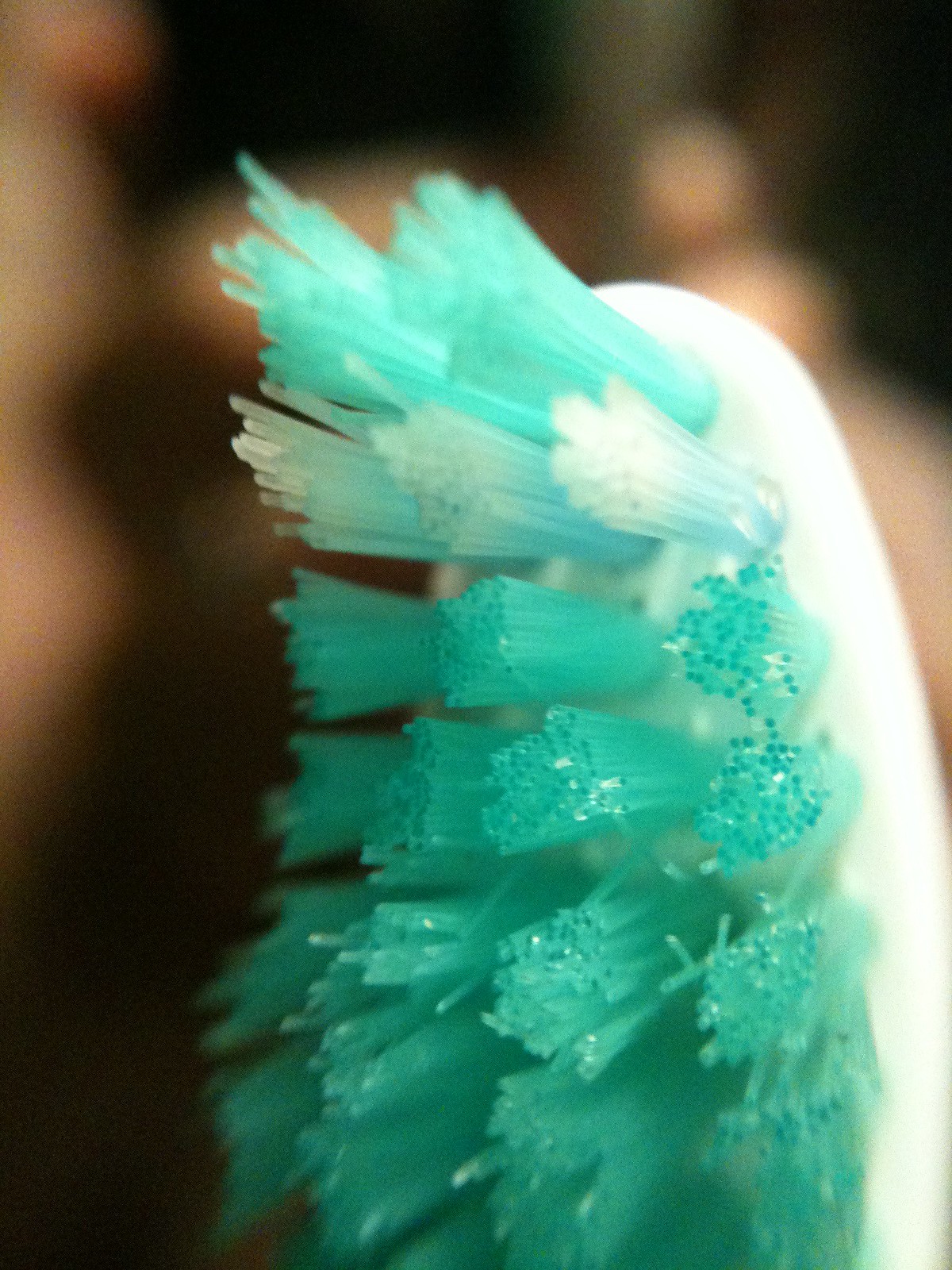The image is an extreme close-up of a white plastic toothbrush head, with the bristles prominently facing forward and taking up about two-thirds of the frame. The toothbrush head is composed of detailed rows of bristles: the top row features two green bristles, followed by a second row containing three sets of blue bristles that fade to white at the tips. Beneath these are five more rows of solid green bristles, perfectly aligned. The photograph is sharply focused on the toothbrush head, leaving the background a soft, blurry mix of tan, black, and various undefined colors and shapes. The stark white of the toothbrush contrasts vividly with the indistinct background, highlighting the intricate design and hues of the bristles.